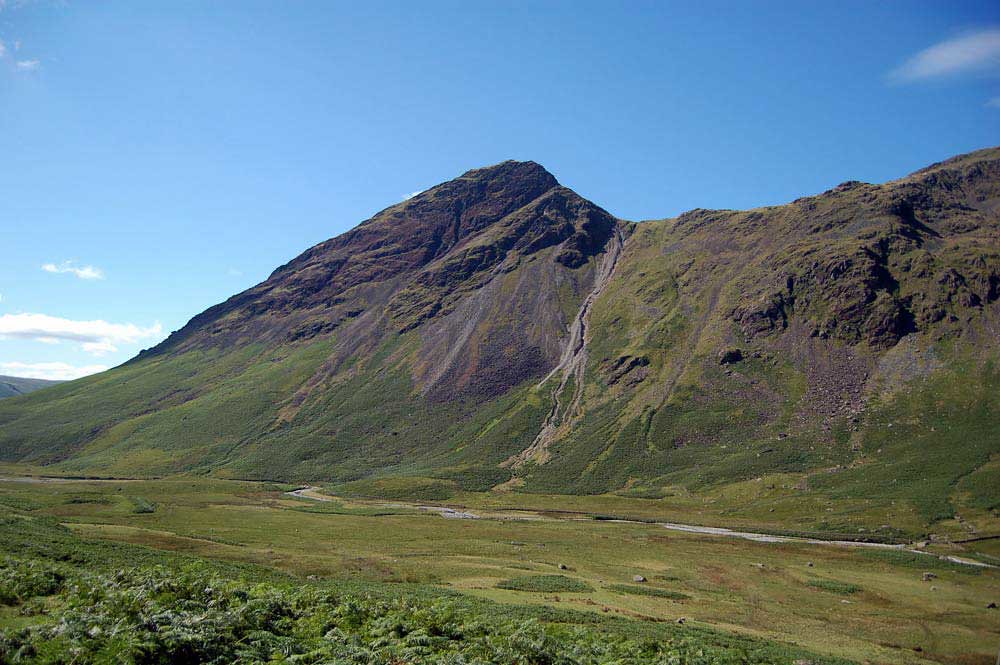This landscape photograph, likely taken in Ireland or a similar setting, captures a craggy mountain that dominates the center and stretches to the right edge. The mountain's lower regions are blanketed with lush green grass and shrubs, transitioning to rocky, dark brown and gray crags as it ascends. The mountain peaks centrally, creating a jagged horizon that dips into a valley on the left before rising and extending horizontally to the right. Shadows accentuate the mountain's rugged texture, especially on the right side. At the mountain's base lies a small, dry riverbed, spanning horizontally from the left to the right of the image, flanked by green grass in the foreground, which turns browner, indicating some dehydration. Above this natural scene, a mostly clear, bright blue sky with minimal clouds—mainly clustered in the upper right and lower left—enhances the overall tranquility and beauty of the landscape. Pathways or trails meander through the greenery, adding a hint of human presence to this serene setting.